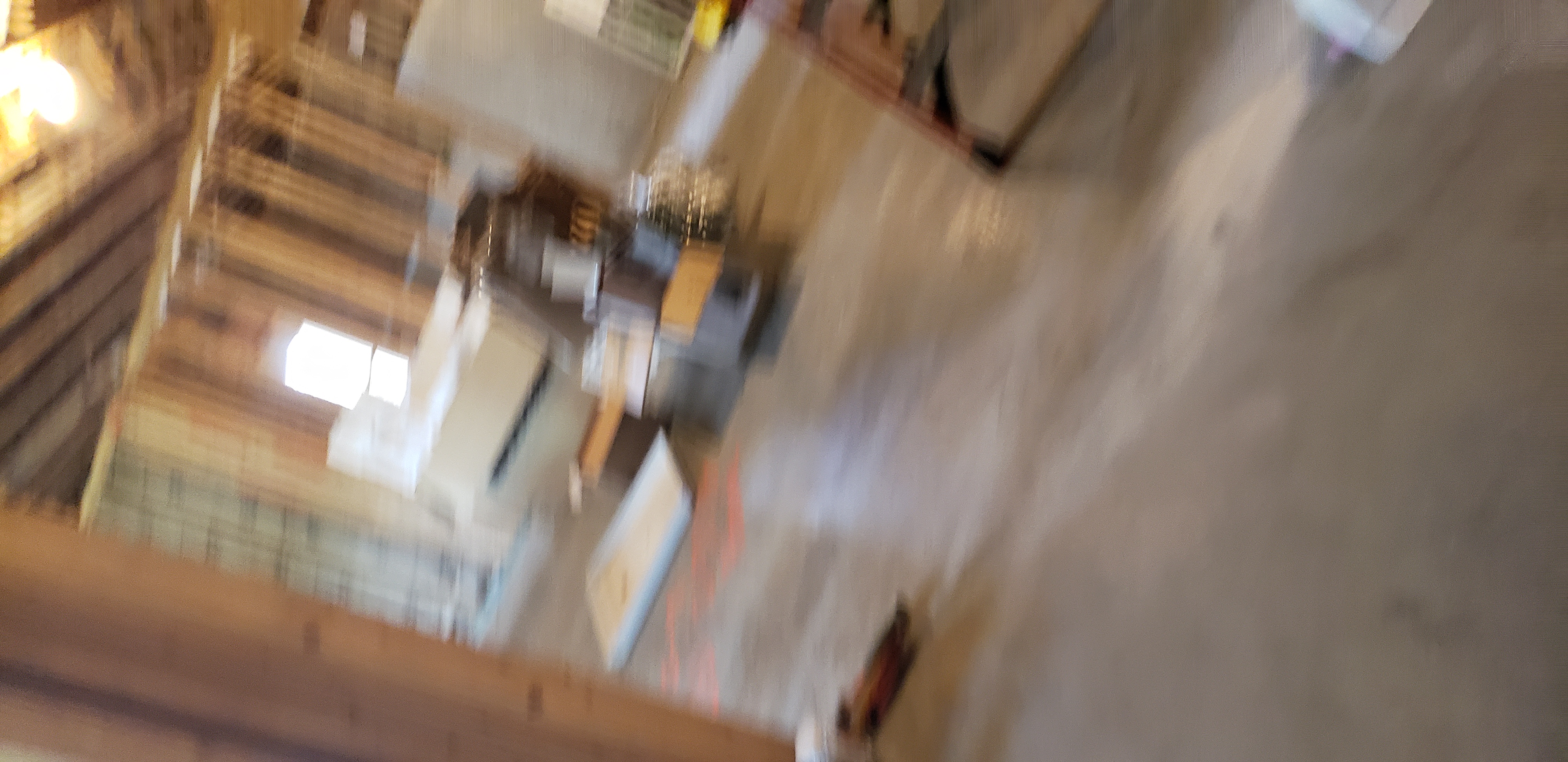This image appears to be a very blurry, vertically-oriented photo, rotated 90 degrees to the right, capturing an active construction site for a house. The foreground showcases a concrete floor, while the middle of the frame prominently features an unfinished wall with a visible wooden frame, featuring gaps between the support pillars. The ceiling structure, composed of exposed 2x4 wooden beams, lacks insulation, but a light bulb is installed and hanging from above. Adjacent to this wall is another section showing installed insulation. In the center of the site, various equipment and materials are piled up, including what seems to be an air conditioner near a partially finished gray wall, and potentially a gray and orange vacuum and a notebook. On the right side of the image, which requires the viewer to tilt their head 90 degrees to the left for proper orientation, there appears to be a darker brown stool or part of a chair. Light filters in from a window on the left, contributing to the overall clarity and detail despite the photo's blurriness.